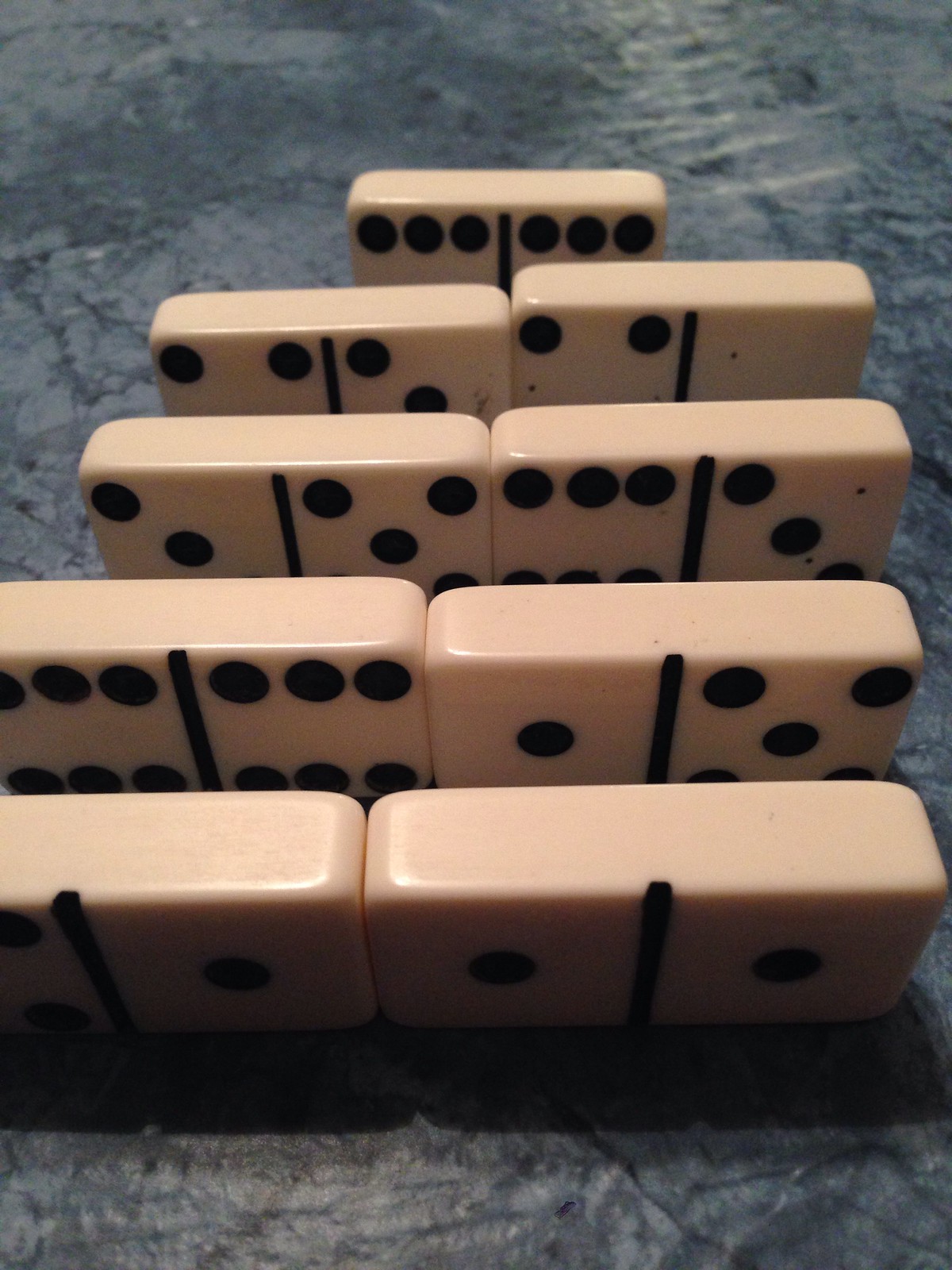This is a colored photograph, possibly taken indoors, featuring a set of white dominoes with black dots and lines, meticulously arranged against a richly textured, blue-patterned background with shades varying from light to dark blue, and touches of black. There are nine dominoes in total, standing on their longer sides in four tightly clustered rows, with each row consisting of two closely touching dominoes, except for one row that has a single domino. 

Starting from the front, the first row has dominoes marked with numbers 1 and partially visible 1; the second row displays 1 and 5; the third row consists of two 6s; the fourth row features 3 and 5; the fifth row presents 6 and 3. In the very back row, a lone domino marked with a 4 is visible, and another adjacent one has markings that are slightly obscured but likely include a 6. Low lighting gives the photo a slightly dim ambiance, enhancing the contrast between the beige dominoes and the intricate blue background.